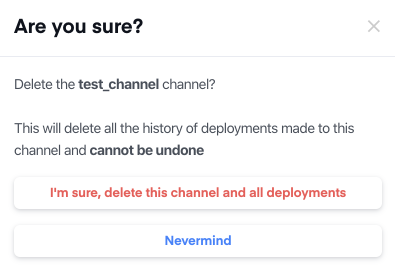This screenshot features a minimalist design with a predominantly white background. Centered at the top in large, bold, black text is the question "Are you sure?" To the far right of this heading, there is a clickable light gray "X" symbol, indicating the option to close or dismiss the prompt. Just below this title, a thin gray line spans the width of the image, separating the heading from the body content.

The body of the prompt contains crucial information in dark gray text. It begins by stating, "Delete the test channel channel." Following a space, the text continues, specifying, "This will delete all the history of deployments made to this channel and cannot be undone." Notably, the phrases "test channel" and "cannot be undone" are emphasized in bold, highlighting their importance.

Beneath this explanatory text, the interface presents two buttons for user interaction. The first button, prominently, in red text, reads "I'm sure, delete this channel and all deployments," signaling a decisive action. The second button, situated at the bottom and featuring blue text, reads "NEVERMIND," providing an option to cancel the action. There is no punctuation following the text on this button, and "NEVERMIND" is entirely capitalized.